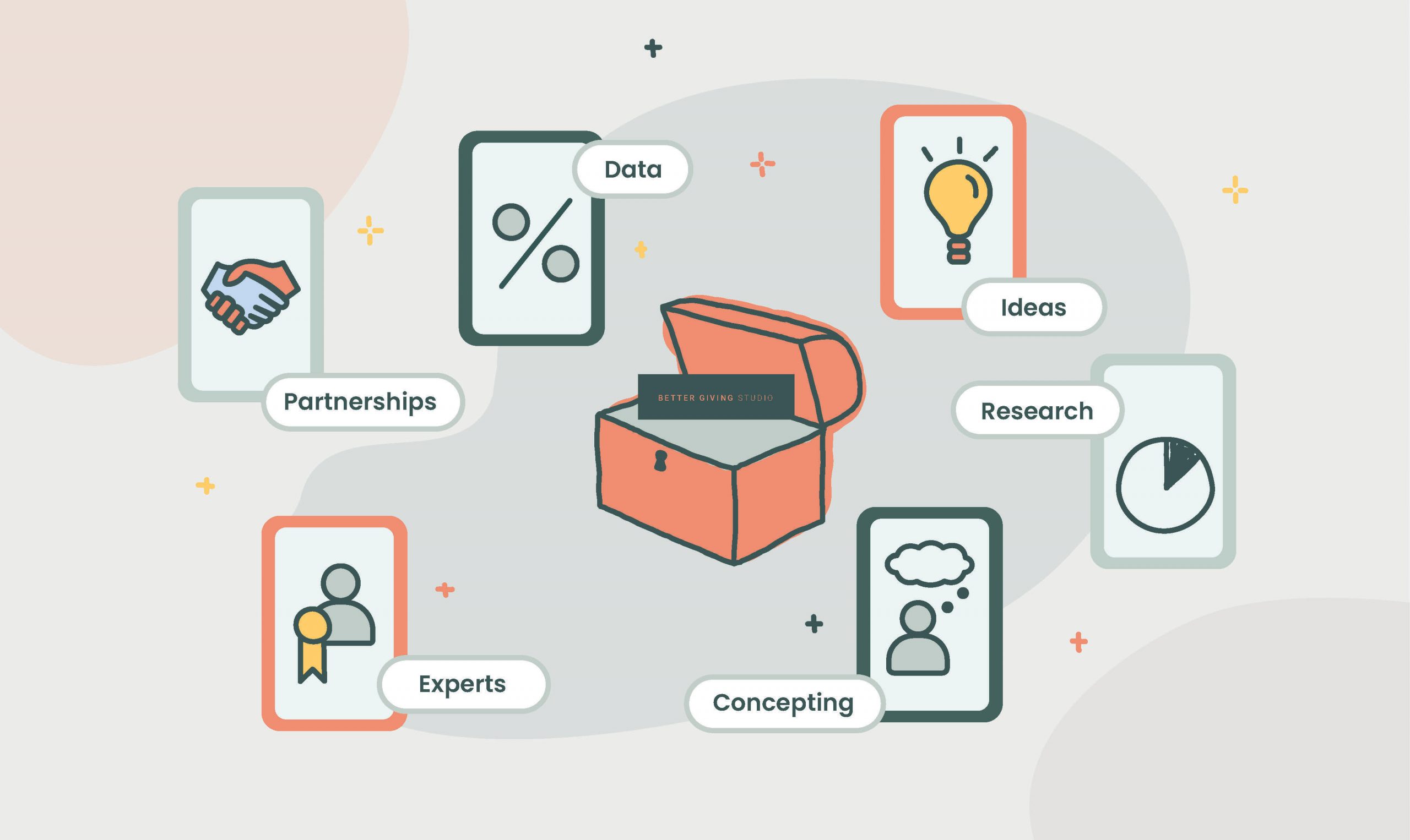This infographic, reminiscent of a slide from a presentation, features a primarily gray, rectangular background accented by a pale pink area in the upper left corner and a darker gray section in the bottom right corner. Scatterings of orange and yellow crosses dot the background, adding a subtle layer of detail. Centered in the image is an open orange treasure chest labeled “Better Giving Studio.”

Encircling the central treasure chest are six rectangular cards with distinct illustrations and labels, akin to playing cards. Starting from the top left, the first card, outlined in green, features two clasping hands labeled "Partnerships." Moving clockwise, the next card outlined in gray depicts a percentage sign, indicating "Data." Following this is an orange-bordered card with a light bulb icon annotated with "Ideas." Next is a card with a gray border showcasing a pie chart, titled "Research." Below this, a green-bordered card illustrates a stick figure with a thought bubble, captioned "Concepting." Finally, an orange-bordered card displays a person with a medal, labeled "Experts."

The muted, pastel hues and simplified illustrations impart a mid-century modern aesthetic to the infographic, making it both visually appealing and easy to comprehend.